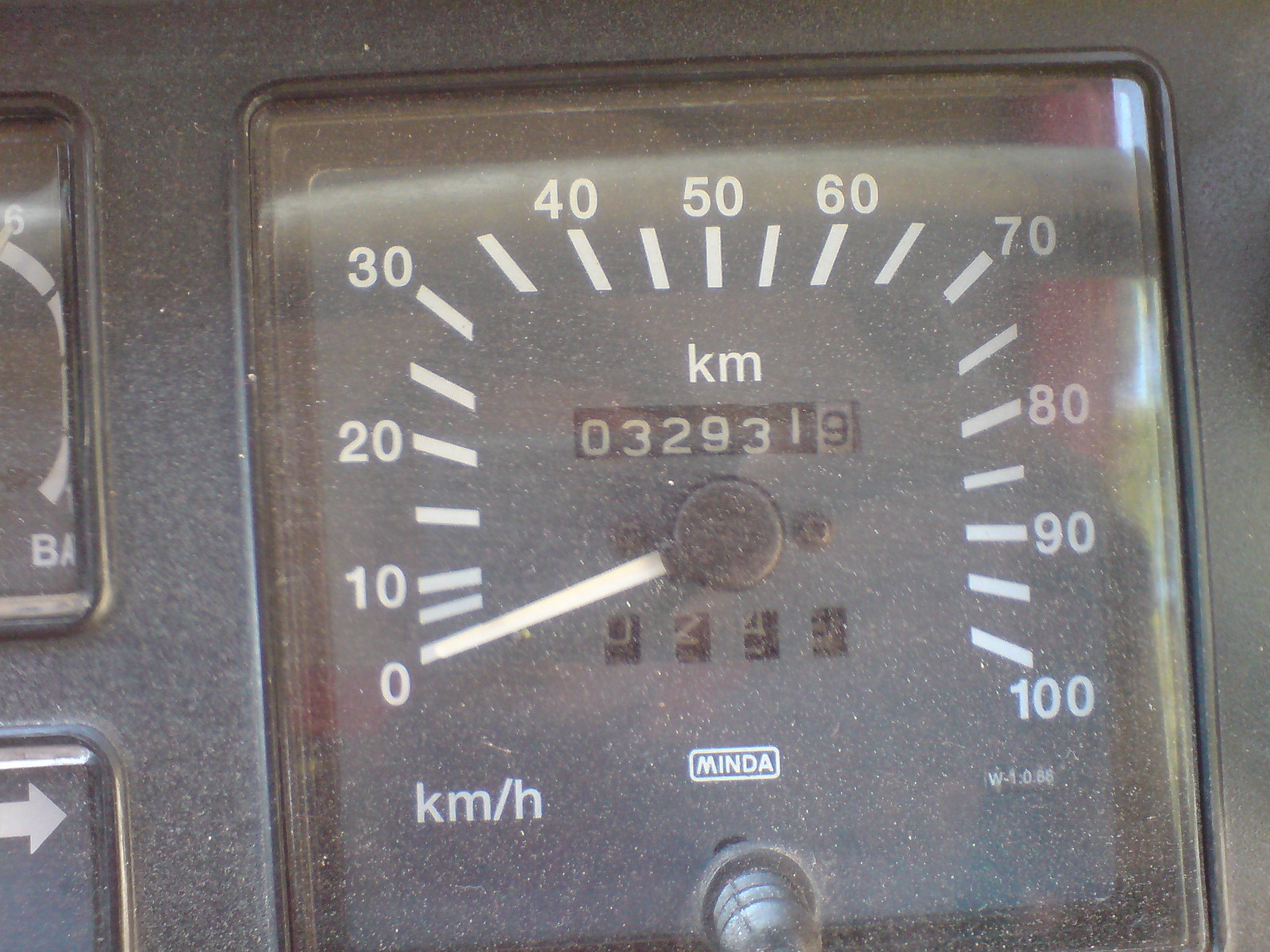A highly detailed close-up of a speedometer, calibrated in kilometers per hour, ranging from 0 to 100 km/h. In the center of the dial, the abbreviation "KM" is displayed in small white letters. Below this indicator, a long rectangular box reveals a rolling odometer, featuring black tumblers with white numbers. The final digit of the odometer appears against a white background with black numbering. The speedometer needle is white with a round black base at its origin, centrally positioned. Four small black squares with white numbers are located below the needle in the center. At the very bottom of the speedometer, "Minda" is inscribed within a white rectangle. The entire dashboard, encased in a transparent plastic cover, exhibits visible dust and specks of dirt. To the left of the speedometer, two additional small square instrument panels can be observed.